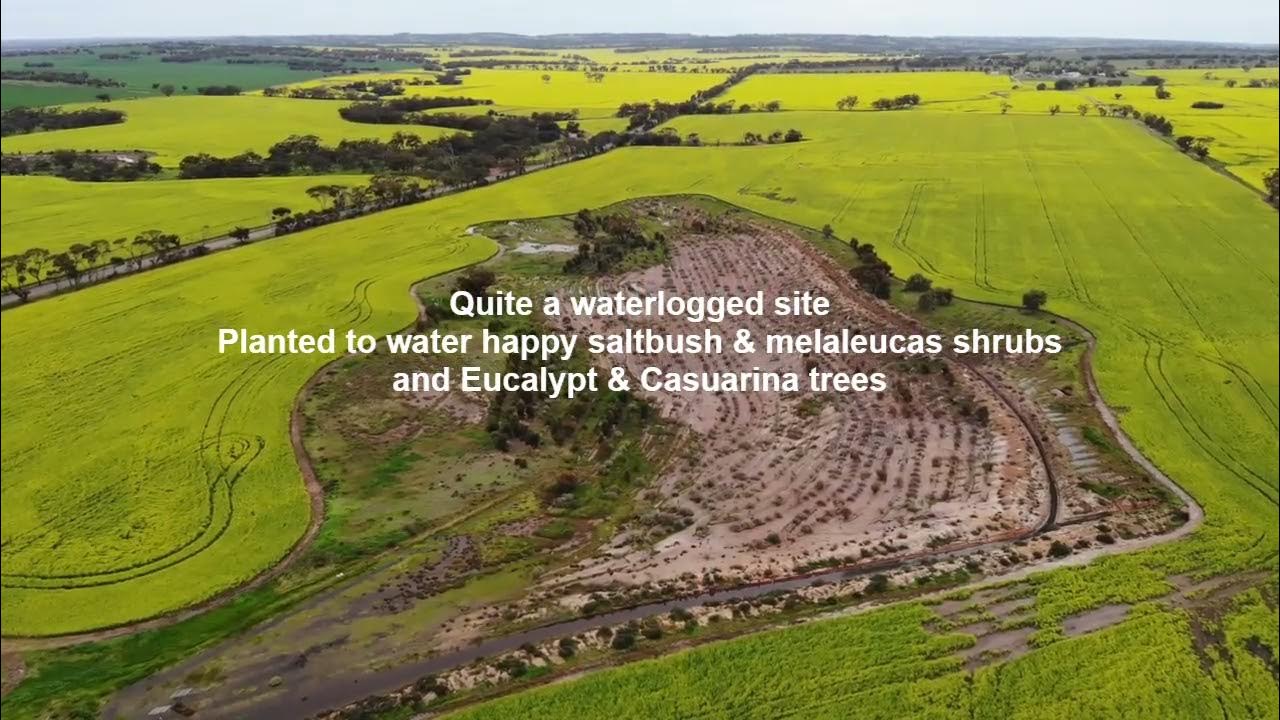This is an aerial photograph depicting an expansive, manicured green field, suggestive of a farming area. The image has a horizontal rectangular orientation, offering a broad view of the terrain. Prominently, on the left side of the image, a tree-lined road stretches into the distance, contributing a structured element to the natural landscape. The majority of the field is covered in light green grass, contrasting with a large centrally located, browned-out area reminiscent of a mud hole. Sparse patches of tiny, struggling shrubs are visible within this desolate zone, indicating possible reforestation efforts. In the background, thin rows of dark green trees and small hills rise, underlining the scope of the area and concluding with a wash of distant blue sky. Overlaying the browned-out section, white text reads, "quite a waterlogged site, planted to water happy saltbush, melaleucus shrubs, and eucalypt and casuarina trees," suggesting an attempt to rehabilitate this swamped area with specific resilient vegetation.